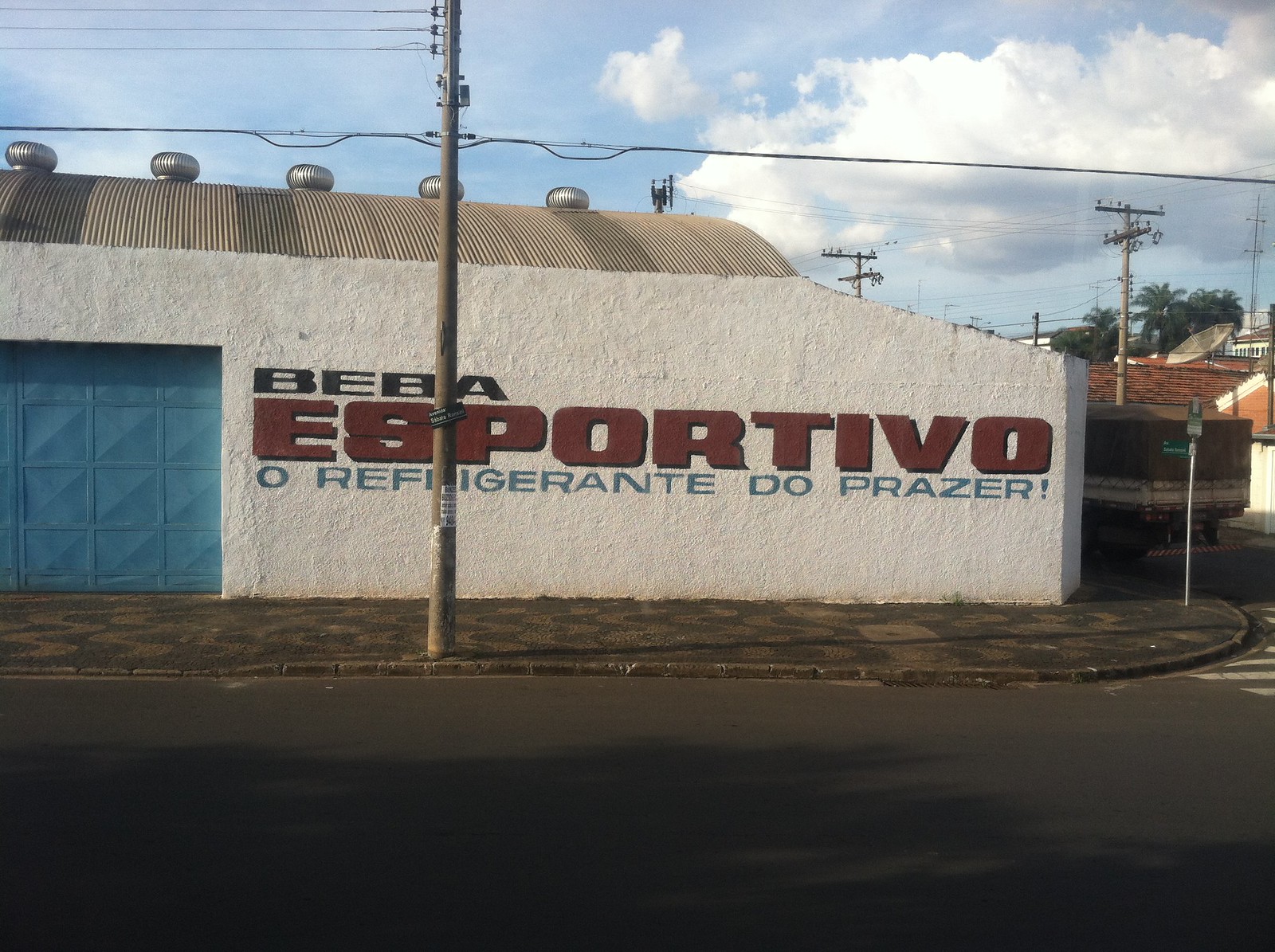The image presents an outdoor scene featuring a building and a roadway. Predominantly, a brown-colored roadway stretches across the bottom of the image, adorned with dark shadows presumably cast by nearby trees. Adjacent to the road is a curved sidewalk sporting hues of brown and black, which seamlessly curves around a corner. Notably, a street sign stands on the right-hand side of the image, while a light pole is situated near the middle on the left. 

Foregrounding the scene is a white building with a stone wall and a beige roof. This building prominently displays a large blue garage door on its left side. Emblazoned on the building are the letters "B-E-B-A" in black, followed by "E-S-P-O-R-T-I-V-O" in bold red letters. Beneath this, smaller blue lettering spells out "Oh, Refrigerante do Prazer!" with an exclamation point. 

In the distance, the image captures houses on the right side and a vibrant blue sky overhead, decorated with a puffy white cloud in the upper right corner. The scene is accentuated by the presence of trees and power lines, contributing to the overall impression of a sunny day.